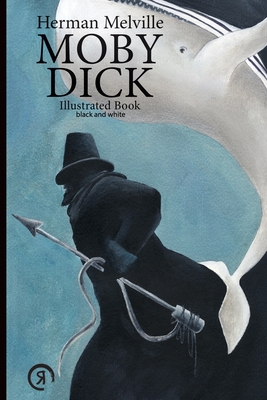The image depicts the cover of the illustrated book Moby Dick by Herman Melville. The cover showcases a dramatic scene featuring a hooded and shadowy figure, likely Captain Ahab, who is holding a harpoon with a wire or cord attached. Although the interior illustrations are rendered in black and white, the cover itself is adorned with color. The background is a dark blue, and the great white whale, Moby Dick, is depicted in stark contrast as a white figure. Moby Dick is shown upside down, as though airborne, perhaps symbolizing the tension and impending clash with Captain Ahab. The captain appears poised to strike, accentuating the intense hunt between man and whale. The illustration highlights the elusive and formidable nature of Moby Dick, capturing the essence of the epic struggle detailed in the novel.